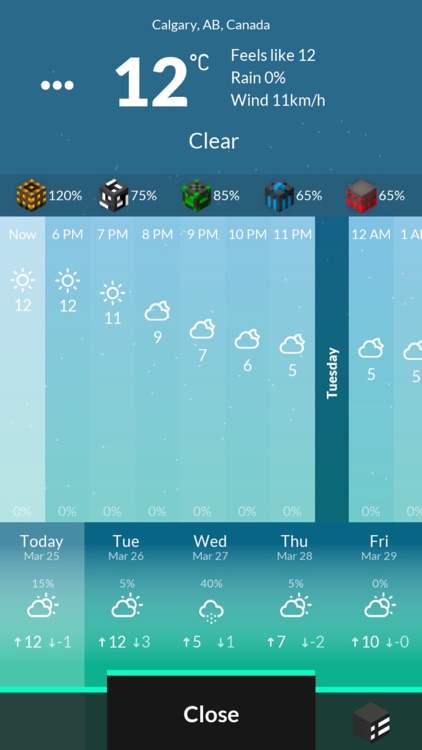This image is a cell phone screenshot displaying a weather application for Calgary, AB, Canada. At the top, a dark aqua blue rectangle features the location name "Calgary, AB, Canada" centered in white text. Below this, the current temperature is prominently displayed as a large, bold, white number "12"°C. Underneath the main temperature reading, additional weather details are provided in three lines of white text: "Feels like 12," "Rain 0%," and "Wind 11 km/h." 

To the right of the temperature, the word "Clear" appears in white text, indicating current weather conditions. Adjacent to the main temperature display, on the left side, are three horizontal white circles representing an ellipsis. Just below, a menu bar presents a series of icons with associated percentages, including values of 120%, 75%, 85%, 65%, and 65%.

Further down, an hourly forecast is laid out in horizontal rectangles with vertical partitions, detailing the weather from "Now" through "6pm," "7pm," "8pm," continuing until "1am." Directly beneath this, another horizontal rectangle displays the weather forecast for the upcoming days: today, Tuesday, Wednesday, Thursday, and Friday, along with corresponding dates, weather icons, and temperature predictions, all in white text.

At the very bottom of the screen, a black rectangle spans across the width of the display, topped by a thin lime green line. Centered within this is a prominent black "Close" button, indicating an option to exit the application.